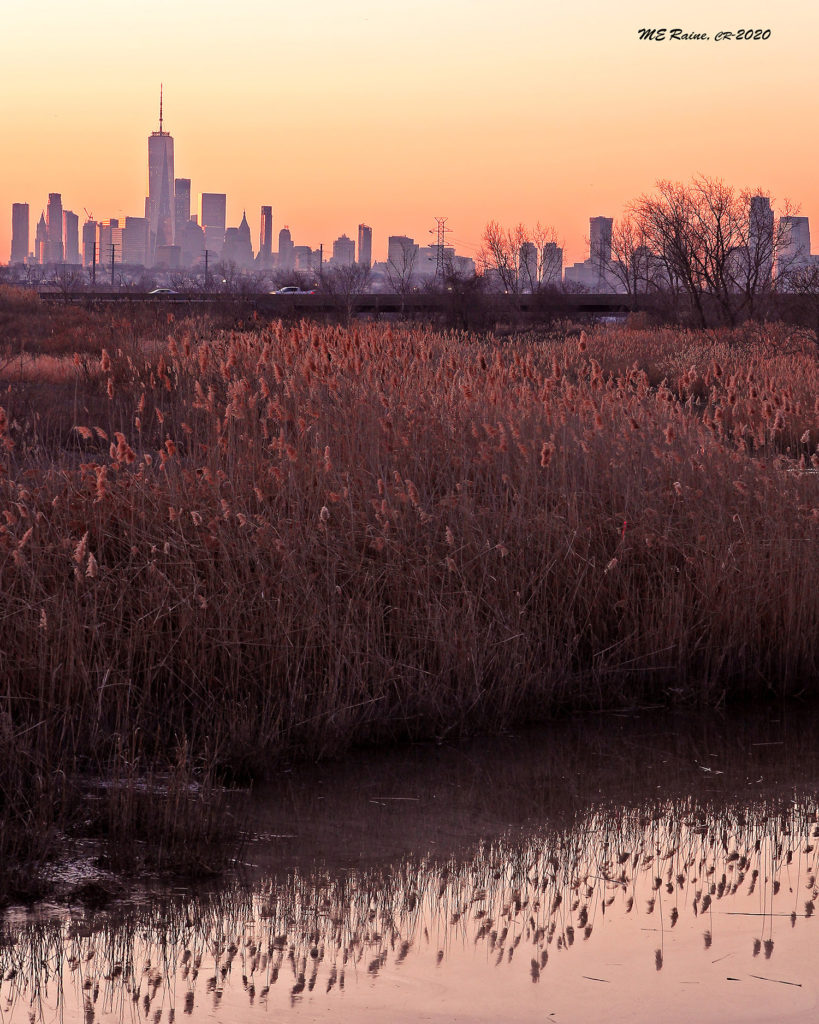The photograph in portrait mode captures a beautiful post-sunset scene. The sky transitions from pink to orange and yellow hues, providing a soft, colorful backdrop. The top right corner of the image features the text "MERAINE CR/2020." Below the sky, the silhouettes of city buildings, including one with a prominent antenna, are visible against the horizon. Some of these buildings exhibit a faint purple and orange glow. Just beneath this urban skyline, an overhead highway is busy with cars traveling leftward. 

The lower half of the image transitions into a picturesque mix of natural elements. The midsection showcases a vibrant swampy field filled with red and orange flowers, dark stalks, and patches of tall grass. Adjacent to the right side, clusters of trees add to the scene's depth. This rich tapestry of flora continues downwards, eventually giving way to a calm, reflective body of water. The water mirrors the vivid colors of the sky and the various plants, creating a harmonious and serene composition. The overall effect is a blend of urban and natural beauty, wonderfully capturing the essence of dusk.